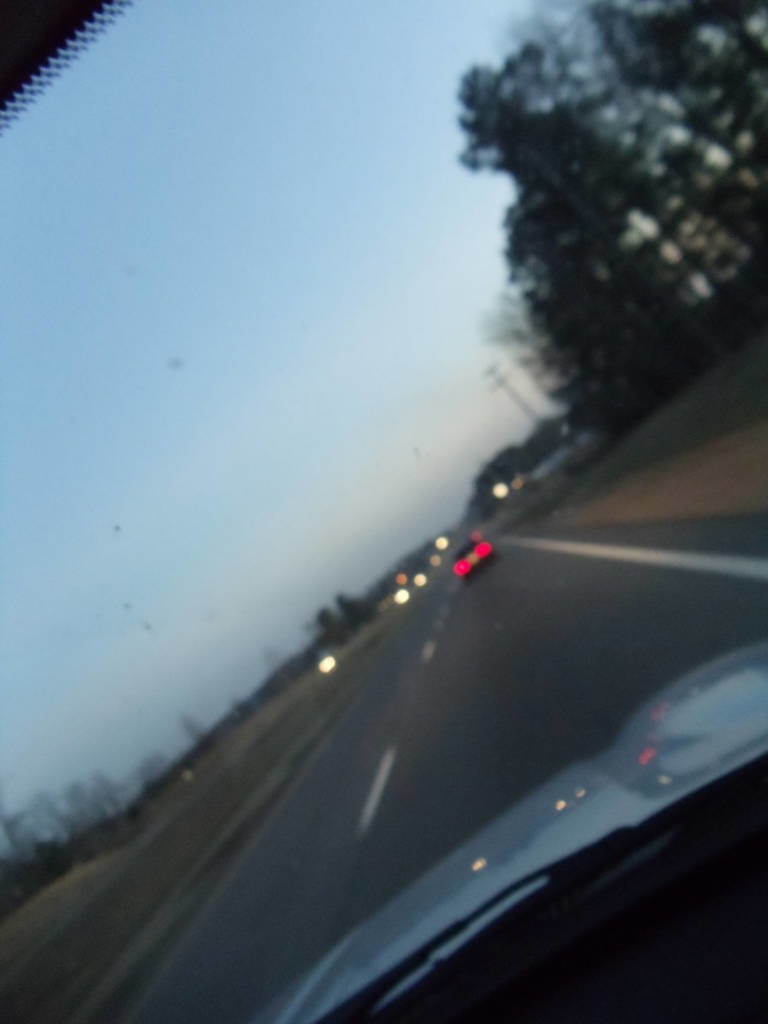This close-up photograph captures the interior of a car, likely in gray or blue hues, though the exact color is indiscernible due to the subdued lighting, suggesting it is either dusk or early evening. The view focuses on the dashboard, revealing limited visibility of the car’s hood and the road beyond. The driver is traveling on the right side of a tree-lined road, with towering trees flanking either side, immersing the scene in a natural, forested environment. Ahead, a single car is visible, albeit out of focus, with illuminated red taillights piercing through the dim surroundings. The sky above is a gradient of soft blue, hinting at the approaching nightfall, and casting the entire scene in a serene, twilight atmosphere.